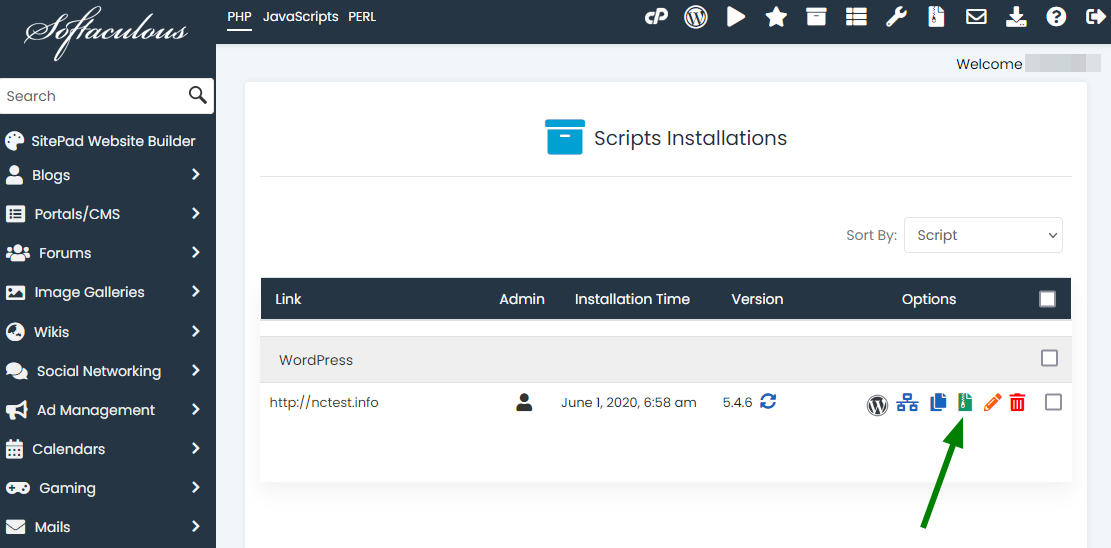This is an enhanced and detailed caption for the image:

"The screenshot depicts the interface of a website known as Softaculous, identifiable by its stylish cursive script logo located in the upper left corner. Running vertically along the left sidebar, there are various categories listed against a dark grey background, featuring white text. These categories include: SitePad Website Builder, Blogs, Portals, Forums, Image Galleries, Wikis, Social Networking, Ad Management, Calendars, Aiming, and Mails. The main content area of the website is predominantly white, with minimal text. At the top of the page, there is a header labeled 'Script Installations,' and beneath this is a mid-page banner displaying columns titled Link, Admin, Installation Time, Version, and Options. Specifically under the 'Link' column, there is an entry for WordPress corresponding to the URL http://nctest.info, with an installation date and time of June 1st, 2020, at 6:58 am. The 'Options' column features several icons, including a prominently displayed green arrow pointing towards a green icon, though the exact function of these icons remains unclear."